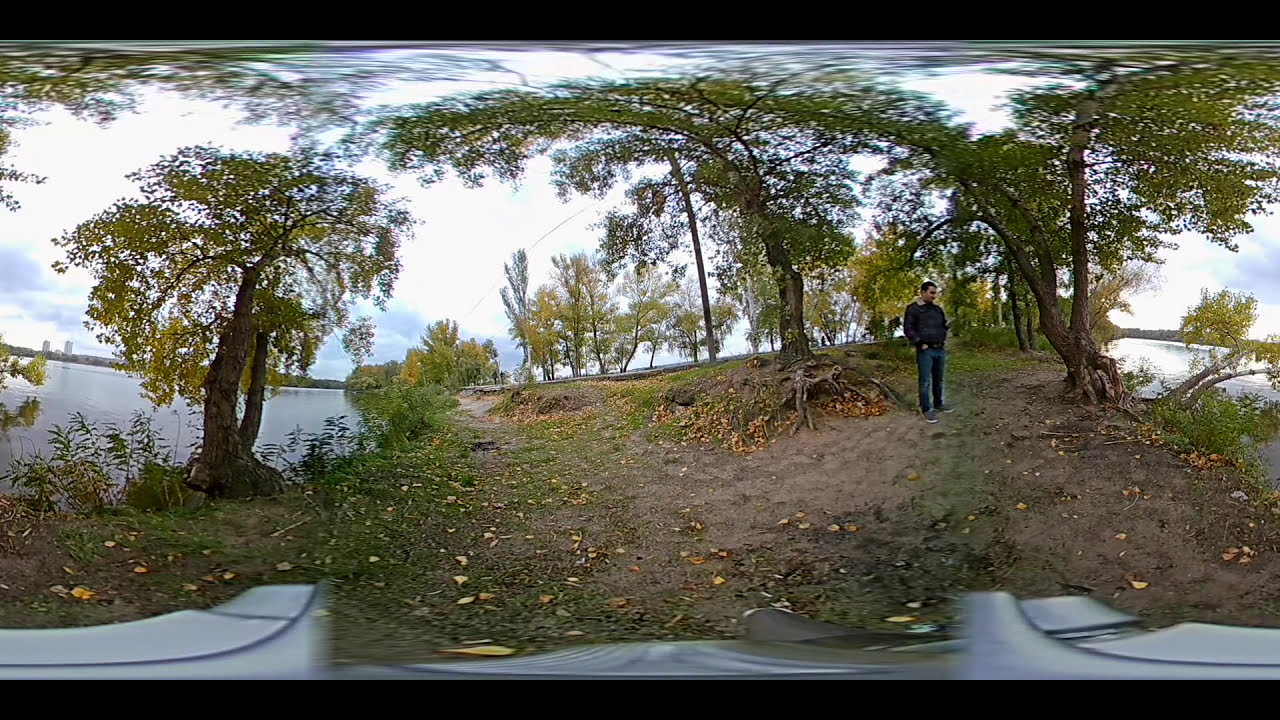In this outdoor panoramic image, a man stands slightly off-center to the right, looking down to his right. He is wearing a dark jacket and blue jeans and has dark hair. The ground is primarily composed of dirt interspersed with leaves, sticks, and small bushes, with very sparse grass cover. In the middle of the image, a prominent tree stands with its roots partially exposed, spreading over the dirt. The tree has green leaves and a brown trunk, and its roots are light brown. To the left and right sides of the image, there are bodies of water, reflecting a pale blue hue from the sky above. More trees, ranging from 12 to 15 feet in height, border these water bodies, with their branches dipping towards both the water and the land. In the background, the sky is a mix of white and blue with a few scattered clouds. The image includes various colors such as black, green, white, gray, brown, yellow, tan, blue, and orange, creating a serene, natural setting in the middle of the day.